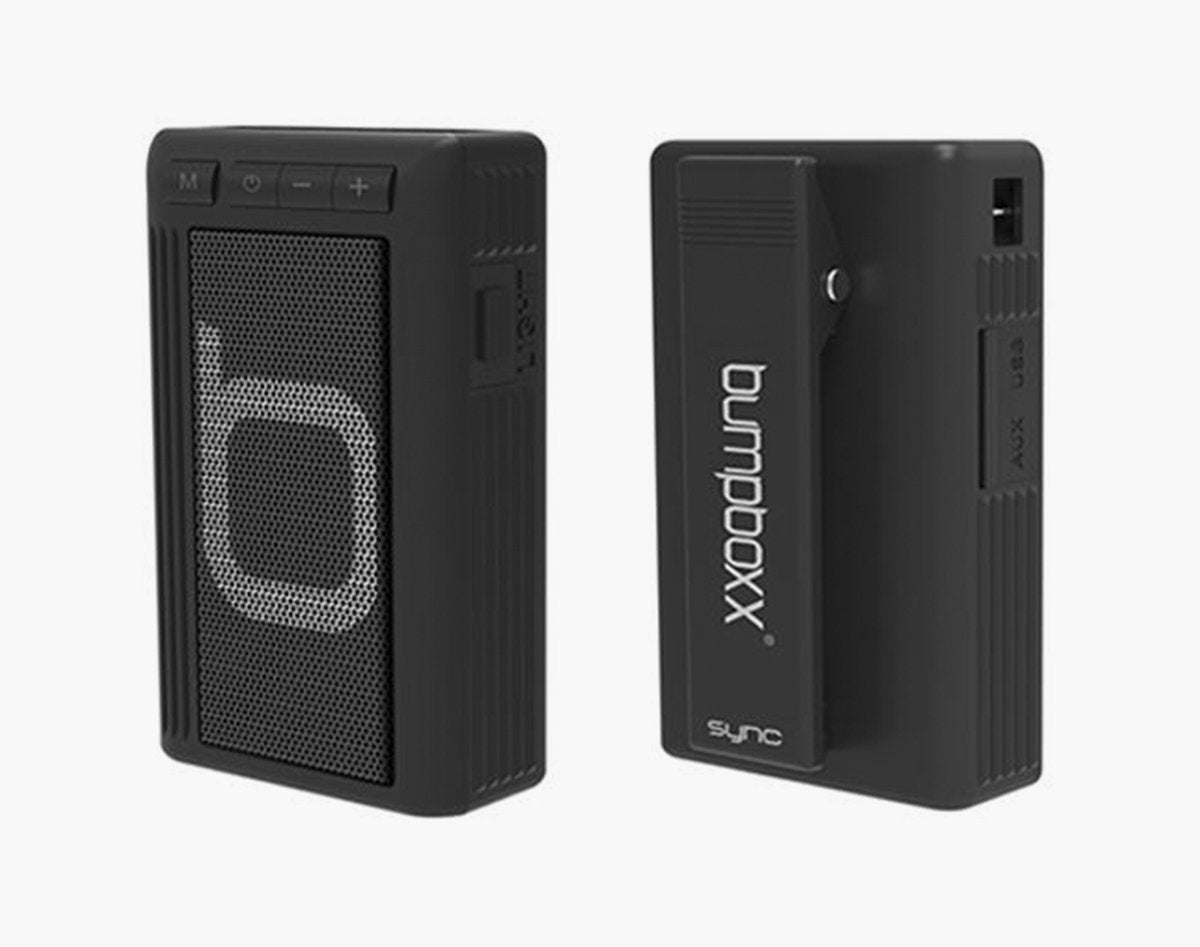This image is a detailed product photo of a small, rectangular, black speaker with two views: front and back. The front view, situated on the left, showcases the speaker grille featuring a white, lowercase letter "b". Above the grille, there are four buttons on the left side: one marked with an "M", followed by buttons for power, volume down, and volume up. A ribbed button is noticeable on the side of the speaker. The back view reveals a belt clip with the words "Bumpboxx" written vertically and the word "Sink" in white at the bottom. The right side view of the speaker shows a slot designed for an aux cable and a small rectangular space near the top, equipped with a silver bar likely for attaching a strap. The device appears short and thick, emitting a modern yet simple design.